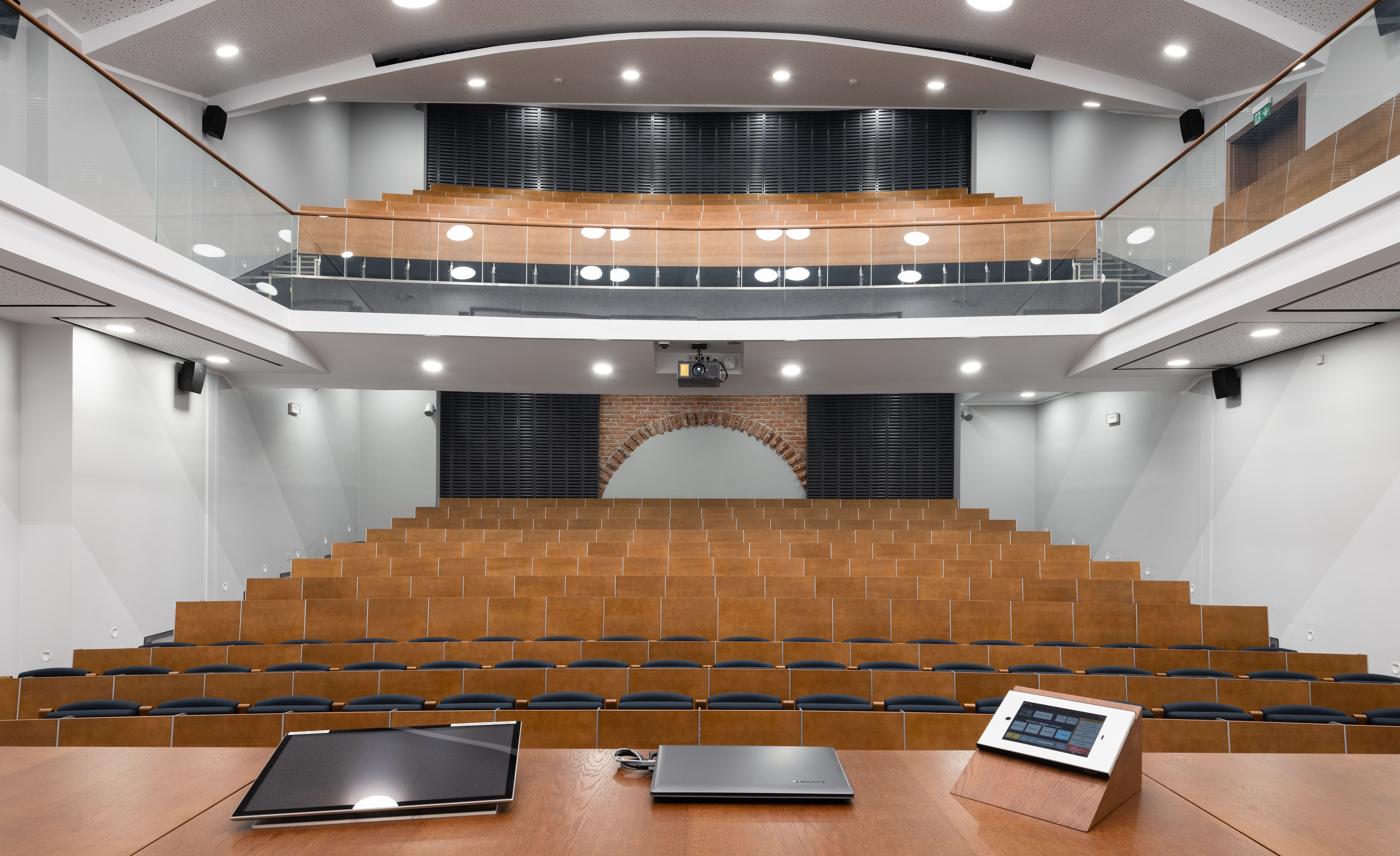This image depicts the interior of a modern lecture hall or auditorium with two levels of seating. The architecture features white walls and ceilings punctuated by numerous small, round recessed lights, enhancing the brightness of the space. The back of the auditorium is characterized by a distinctive red brick wall framed by two indiscernible black objects. The seating, predominantly wooden, is arranged in rows on both levels, with the upper level featuring a glass safety barrier. The stage at the front displays three distinct items: a tablet on the left, a closed silver laptop in the center, and an angled device on the right, possibly a control board. The overall design is sleek and contemporary, accommodating several hundred attendees and ensuring a clear view of the stage from all seats.